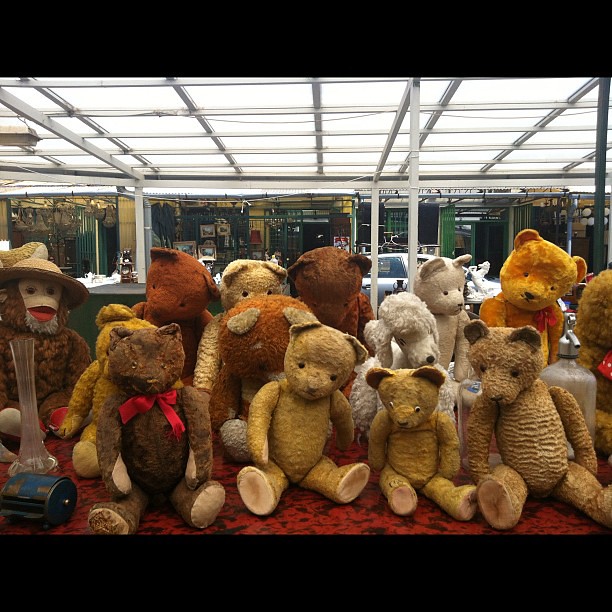This photograph features a large display case filled with various antique stuffed animals and teddy bears, predominantly from the early 20th century. The bears are of different shades of brown, ranging from russet to golden and medium brown. Their worn fur suggests their vintage nature, and their positions indicate they are on display, likely in an antique store or exhibition hall. Sitting on a red fabric surface, most of the animals face the camera, with the exception of a notable happy monkey with a bright red mouth all the way to the left. Among the bears, one in the front stands out with a red tie around its neck, while another, positioned towards the back left, sports a hat reminiscent of Smokey the Bear. There’s also an old glass vase and an indistinct blue cylindrical metal item included in the scene. Above them is a grid of light tiles casting an even glow over the display. The background hints at multiple international shops, lending an exotic flair to this quaint and nostalgic setup.